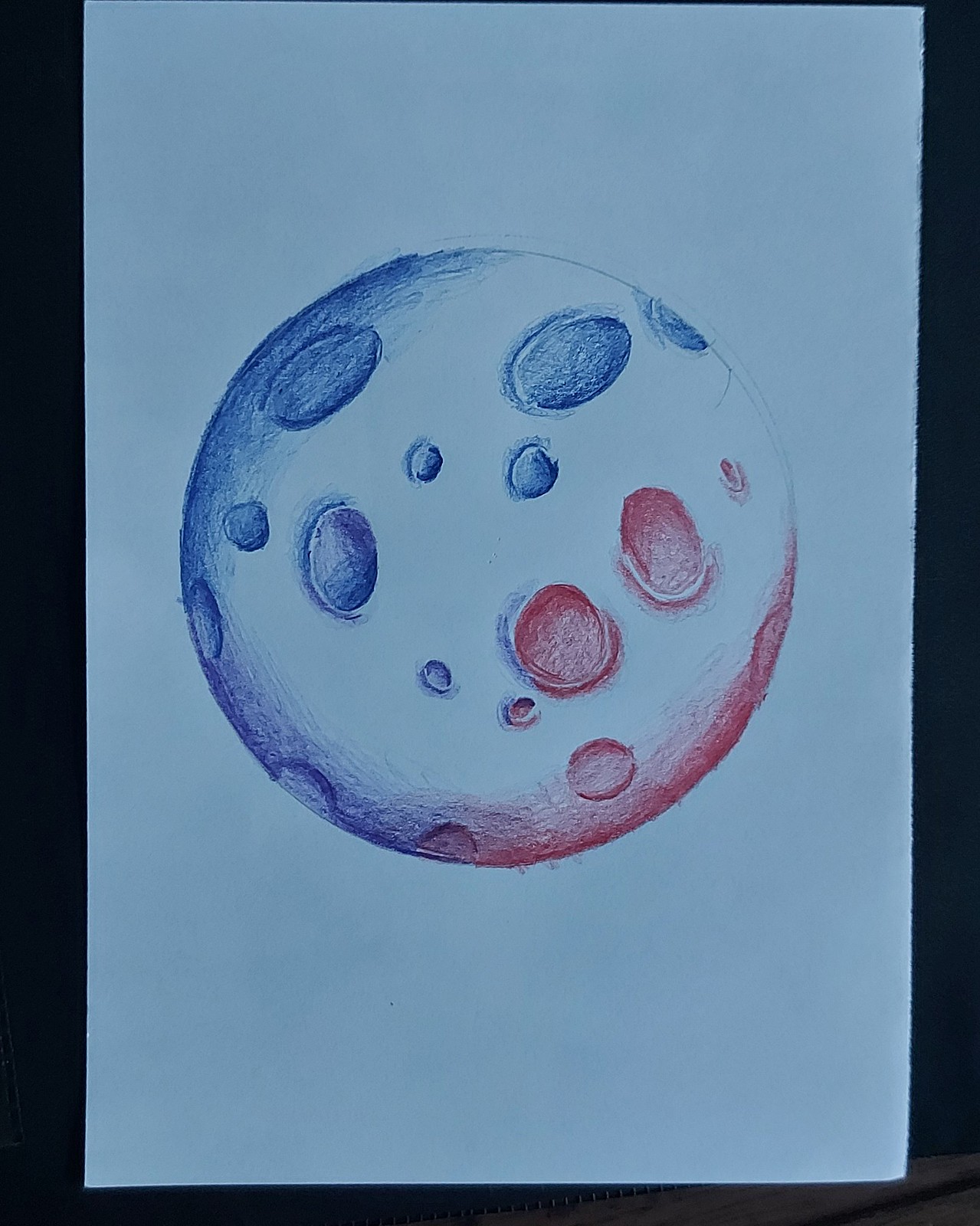This image depicts a spherical object resembling a planet or a ball, primarily white with distinct red and blue accents. The surface of the sphere is characterized by egg-shaped craters in varying sizes, some filled with red and others with blue. The sphere is segmented into three color zones: one with blue edges, another with red, and a third with white, with all sections seamlessly merging together to form a perfect round shape. It rests on a light blue piece of paper, which itself contrasts with the black background, highlighting the vibrant colors and intricate details of the sphere.